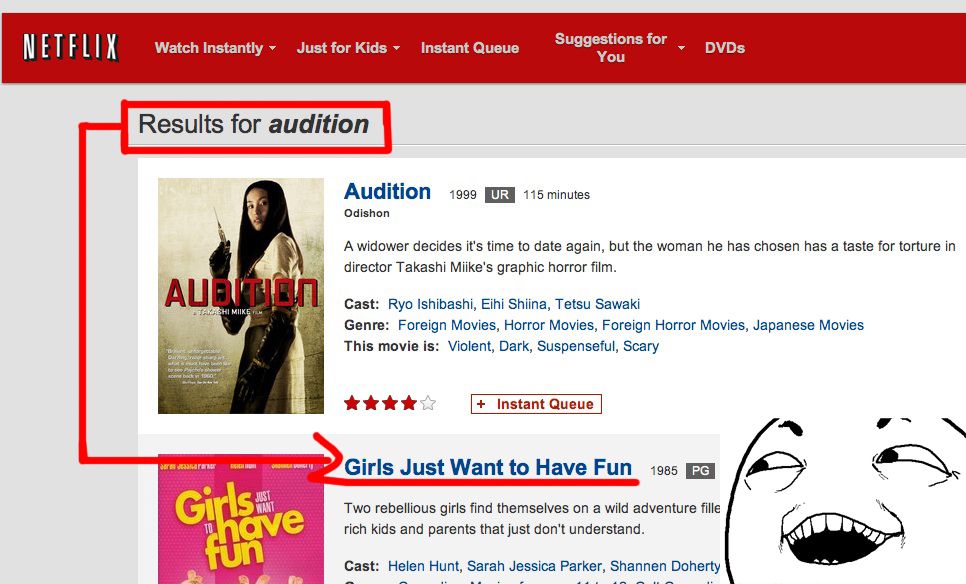The image is a screenshot of the Netflix streaming interface. At the top, against a red background, the Netflix logo is prominently displayed in white text. The navigation menu includes options such as "Watch Instantly," "Just for Kids," "Instant Queue," "Suggestions for You," and "DVDs."

Below the menu, within a red rectangle, black text reads "Results for Audition." An image accompanies the title, featuring a woman of Asian descent holding a needle with a sinister expression on her face. The movie title "Audition" is written in bold red text alongside a brief description: "A preview of the movie from 1999 at 115 minutes. A widower decides it's time to date again, but the woman he has chosen has a taste for torture in director Toshiki Mike's graphic horror film."

Underneath this, another movie titled "Girls Just Want to Have Fun" is showcased. The background is pink, and the synopsis reads: "Two rebellious girls find themselves in a wild adventure filled with rich kids and parents who just don't understand." The artistic contrast and detail in the depiction of both movies highlight the diversity of genres available on the platform.